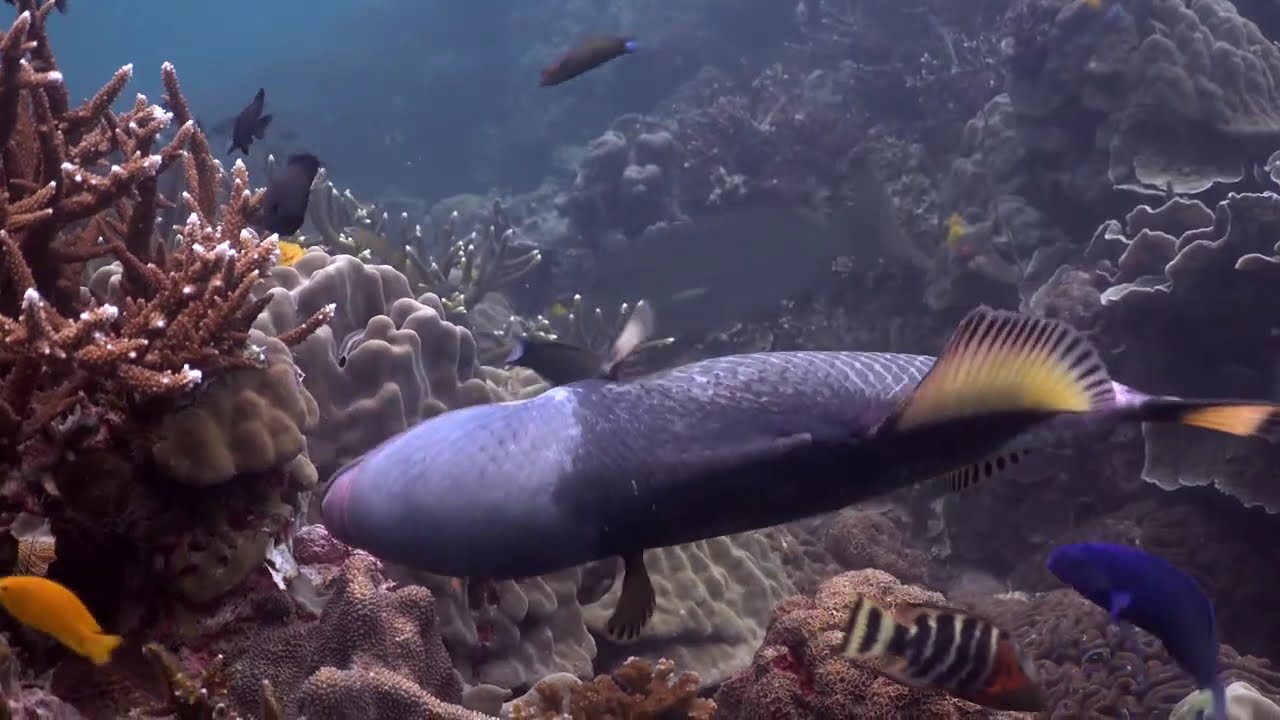This underwater graphic image features a close-up of a very large, vividly colored fish with its head facing the camera and its tail angled towards the upper left corner. The fish has striking details: a purple head with an area around the eye in yellow, an open mouth displaying two prominent white teeth, and a pattern of yellow and black stripes along its body. The section near its belly features a sunbeam design with gold rays emanating. Its fins are yellow with black triangles, and the tail fin is a blend of purple, black, and yellow.

Surrounding the fish, the scene includes a variety of sea life and corals. In the top right corner is a prominent red coral with numerous spiny branches. The bottom of the image showcases white coral formations and what appears to be a black plant element emerging from one of the coral pieces. Smaller purple fish can be seen swimming around the main fish, along with what look like flat, pita bread-shaped sea organisms scattered on the ocean floor. The image does not contain any text, emphasizing its intricate and vibrant underwater setting.